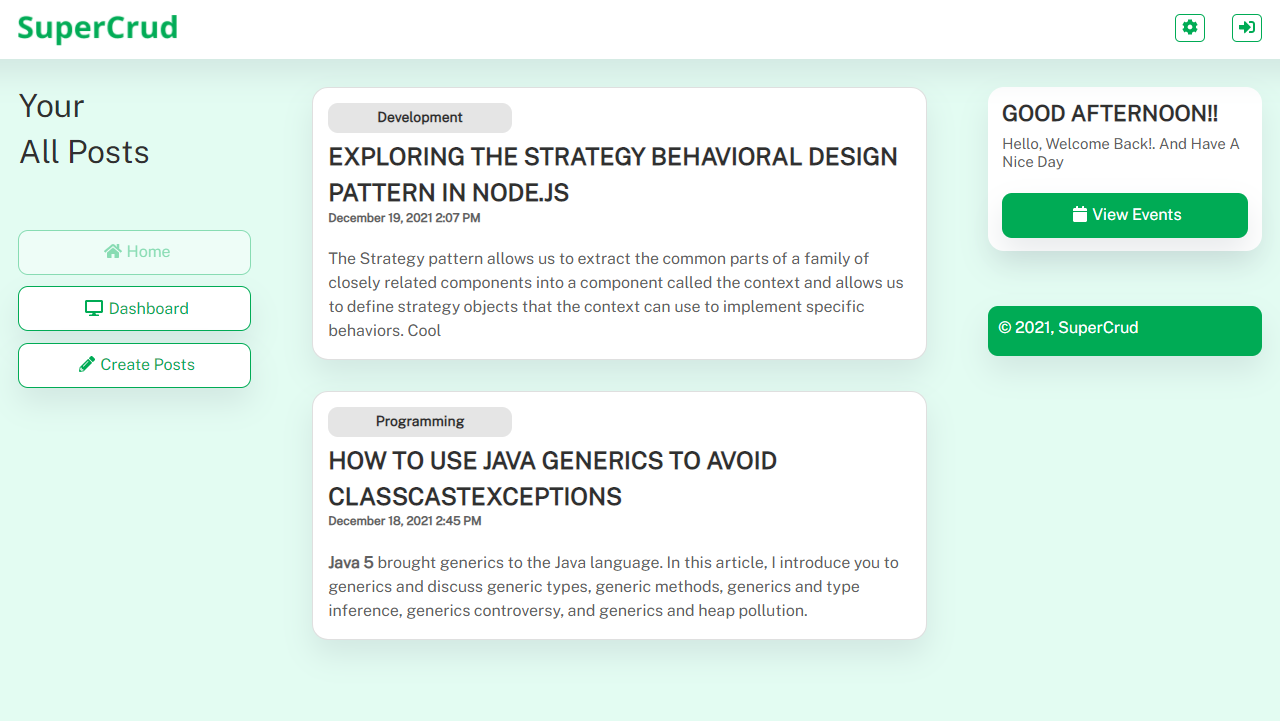The image depicts a screenshot from Supercrud. The recognizable Supercrud logo and brand name are prominently displayed in the upper left-hand corner, rendered in green against a white background. Opposite this, on the right side, there are two distinct icons: a green gear symbol and an arrow pointing to the right with an open bracket to the left.

The main section of the interface contains a blue header with the text "You're All Posts." Below this are navigation options listed as Home, Dashboard, and Create Posts. The Home option is faintly grayed out, while Dashboard and Create Posts are situated on a white background.

Below the navigation, two separate white sections are visible. 

The top section, marked by a gray tab labeled "Development," contains a post titled "Exploring the Strategy Behavioral Design Pattern in Node.js," dated December 19th, 2021, at 2:07 PM. The accompanying text explains the strategy pattern, detailing how it allows the extraction of common components in a family into a context component, enabling the use of strategy objects to implement specific behaviors.

The bottom section is labeled "Programming" and features a post titled "How to Use Java Generics to Avoid Class-Cast Exceptions," dated December 18th, 2021, at 2:45 PM. The article introduces Java generics, covering topics such as generic types, methods, type inference, the controversy around generics, and heap pollution.

On the right side of the interface, phrases like "Good afternoon," "Hello," "Welcome back," and "Have a nice day" are displayed. Additionally, there are two green tabs: one labeled "View Events" and the other "2021 SuperGrid."

The entire interface layout is designed with clear sections and navigational cues, although the top section's text appears as a run-on sentence, whereas the bottom section is punctuated correctly.